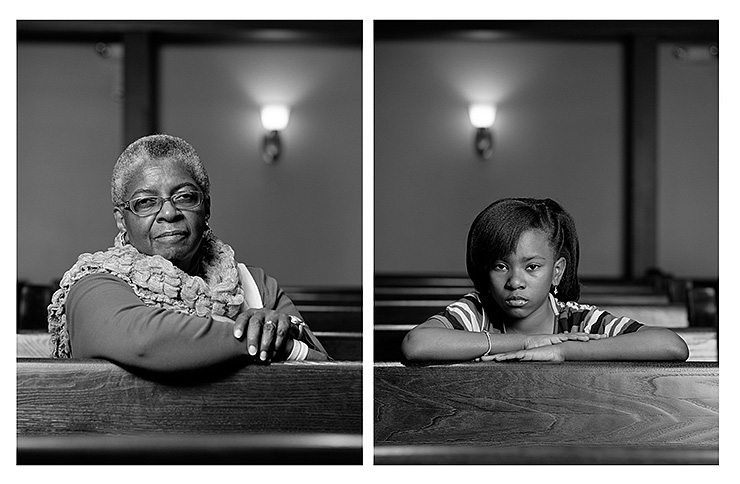The image comprises two black-and-white photographs side by side, capturing a solemn atmosphere within a church. Both panels depict a similar section of the church: rows of wooden pews, white walls, and a lantern-style wall lamp with a white top. The left panel features an older African American woman with short gray hair and glasses. She wears a shawl or furry scarf around her neck and a long-sleeved shirt. Her right arm rests on a pew's back, supported by her left hand, while she gazes thoughtfully at the camera. The right panel shows a young African American girl with shoulder-length, straight black hair. Dressed in a white, gray, and black striped shirt, she too leans her arms on the pew in front of her, mirroring the woman's pose. Both subjects share a similar, contemplative expression, emphasized by the soft glow of the wall lamp behind them, creating a unified and poignant narrative through their mirrored postures and shared surroundings.